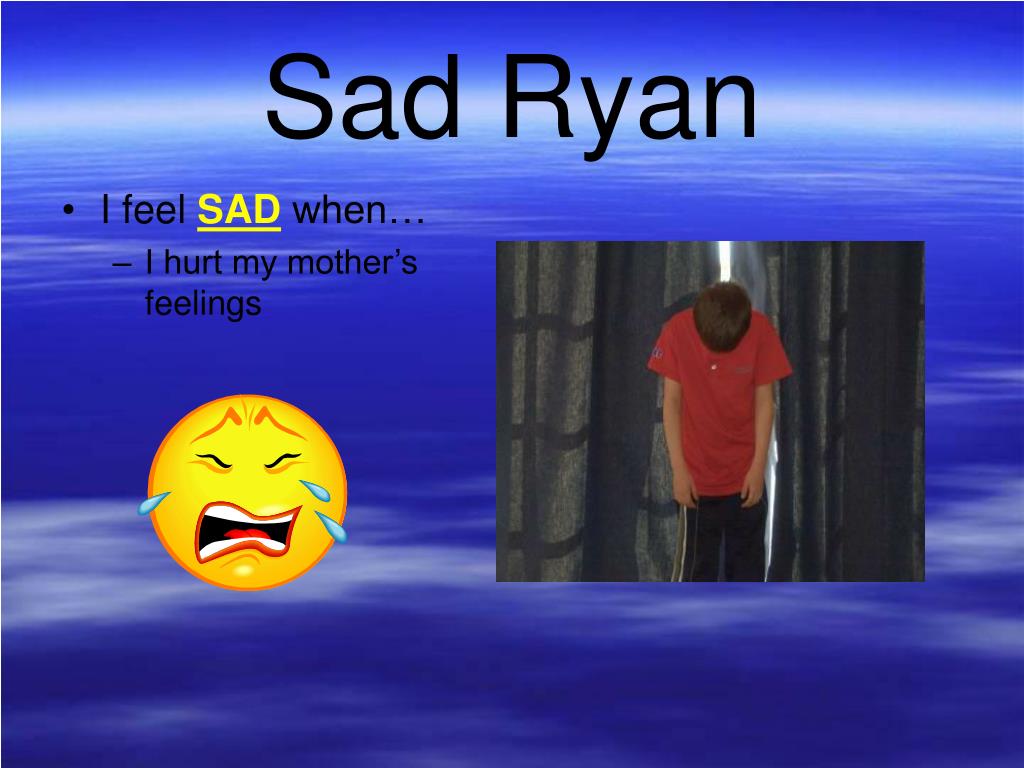In this rectangular poster, the background emulates a sky with blue hues and wispy white clouds stretching horizontally. At the top center, bold black lettering reads "Sad Ryan." Below it on the left side, a bulleted list starts with "I feel" followed by the word "SAD" in capitalized yellow letters, underlined for emphasis. The remainder of the text finishes the sentence, "when I hurt my mother's feelings," all in black. Adjacent to the text is a crying yellow emoji face, complete with blue tears, red lips, and a sorrowful expression. 

On the right side of the poster, a square photo of a young boy named Ryan is inset against a background of gray blinds. Ryan is wearing a red short-sleeve shirt and dark track pants, his head hanging down, obscuring his face, while his arms dangle despondently by his sides. The image poignantly captures his regret and sadness.